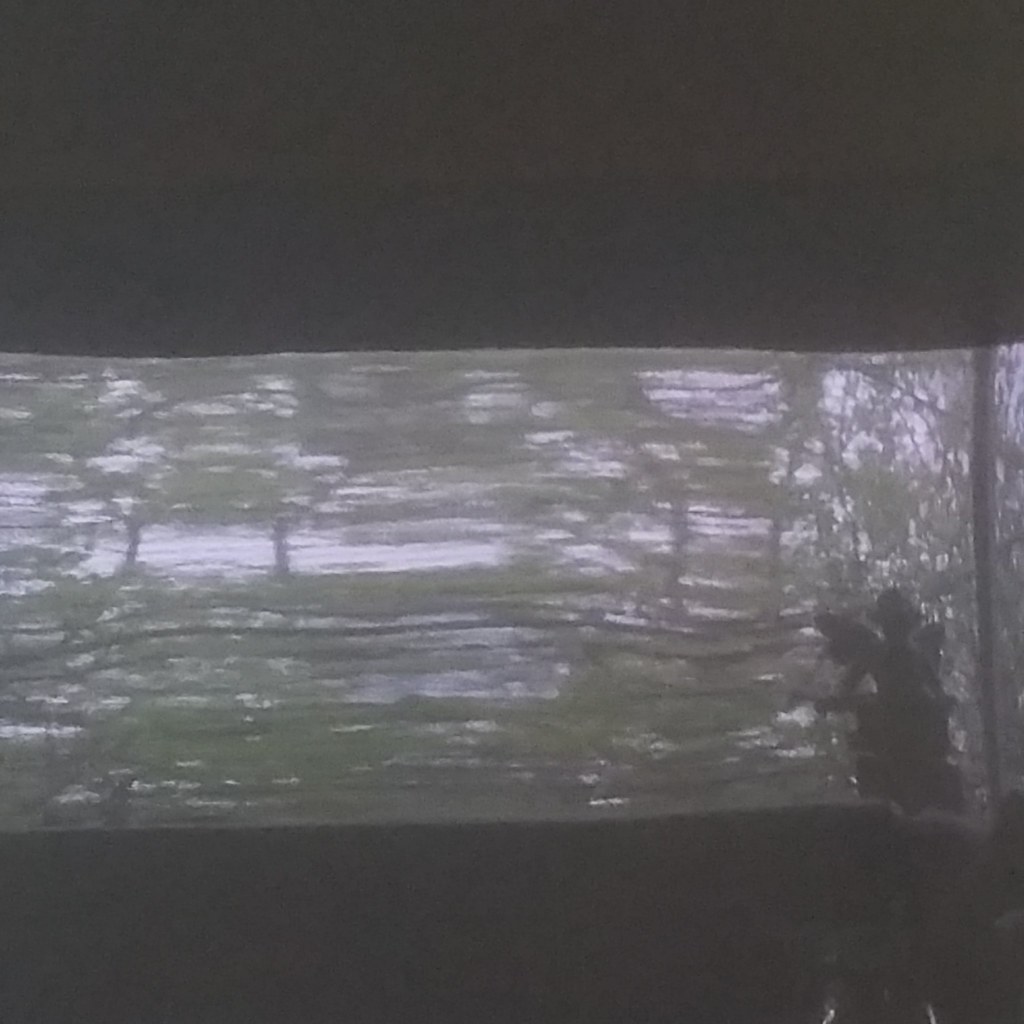The image appears to be a very blurred and smeared projection of an outdoor scene, possibly through a window. It is distinguished by a clear rectangular outline in the center, surrounded by dark areas at the top and bottom that almost frame the scene, possibly resembling the borders of a window or a distorted film still. The middle section is dominated by a blend of trees, where the green leaves merge together against the darker brown trunks. In the upper right, the branches and leaves are slightly more distinguishable against a sky that seems to mix grayish-blue and white hues. The lower right corner features a distinctive, shadowy shape with a boxy bottom and an intricate top design, which could be interpreted as a statue or perhaps a figure reminiscent of a gargoyle. The scene's background on either side of the rectangle is dark, contributing to the overall obscured and dreamlike quality of the image.